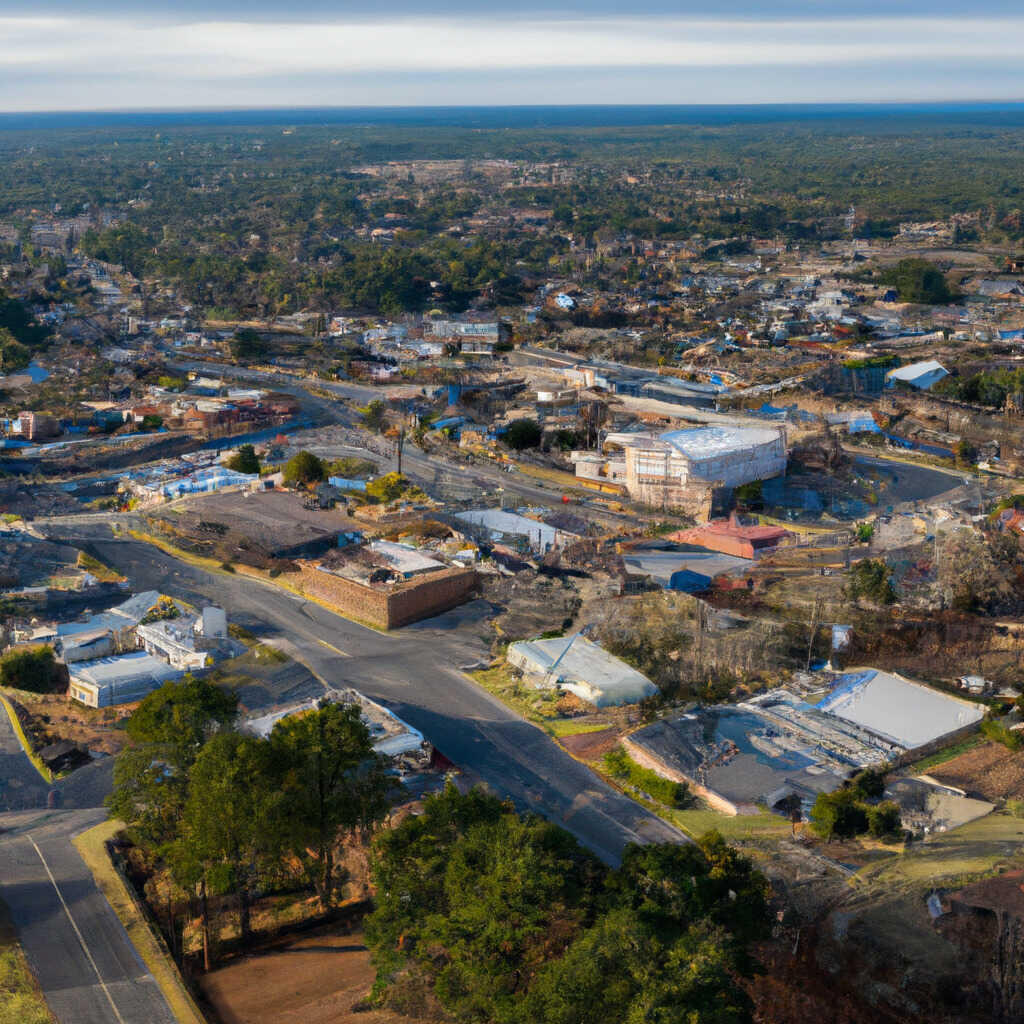This aerial photograph captures an expansive view of a sprawling town stretching to the horizon under a cloudy sky. Dominated by a mix of green lawns and dense trees intertwined with numerous buildings, the landscape gives the impression of a suburban or working-class community, more flat and likely situated in the Midwest or South. The central area of the image showcases significant construction activity, with tall trees interspersed between the roadways. Visible residential neighborhoods comprising both scattered homes and buildings extend into the distance. Key landmarks include a stadium-like structure and a building resembling a school, nestled among the sections of city blocks. Roads crisscross throughout, some with cars visible, weaving a network across the verdant townscape, accented with fields and various green spaces.